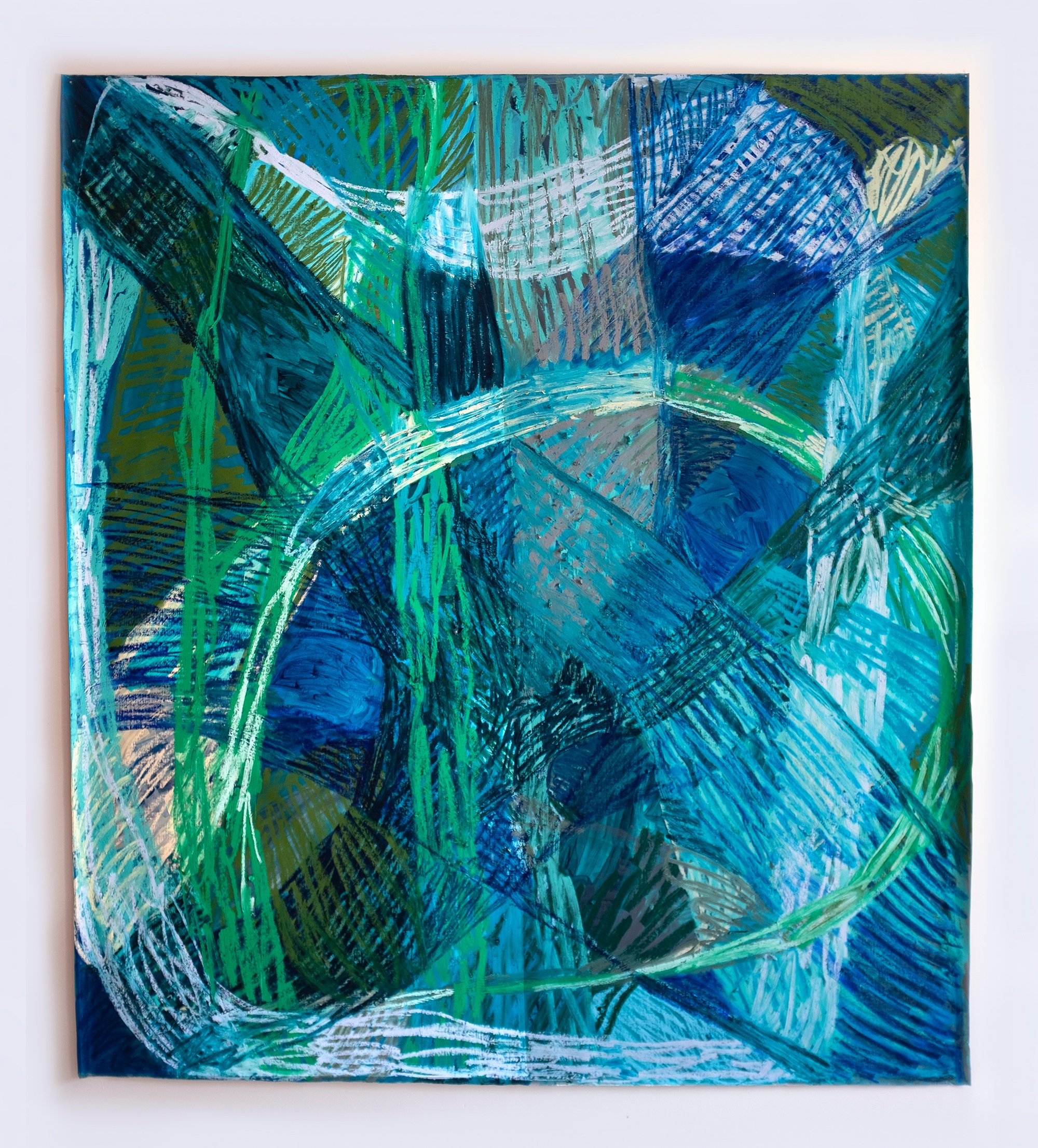The image is of an abstract painting set against a white background and framed within a rectangle. The painting is a dynamic interplay of colors including blue, green, white, beige, yellow, and black, with hints of light blue and grey. The composition features a mixture of intricate cross-hatched and jagged lines, overlaid in various places, creating a sense of organized chaos. Dominant throughout the piece is a thick blue line that runs vertically through the center. Swirls of color meander in and out, with lighter tones of white streaking in almost circular patterns, adding a certain rhythm to the visual narrative. Though busy and complex, the layered patterns and scratch-like lines create an aesthetically appealing and thought-provoking piece, capturing the essence of abstract art where every line and color invites personal interpretation.